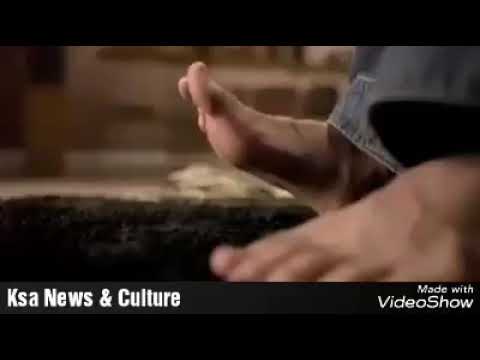This image captures a close-up of a pair of light-skinned feet, positioned on a dark rug or carpet. The left foot is flat on the ground, while the right foot is raised with only the heel touching the floor, possibly suggesting a tapping motion to music. The person is wearing light blue denim jeans. The blurred background reveals indistinct coffee-colored or tan hues and some brown wooden furniture. The image features horizontal black bars at the top and bottom, with text in white font. At the bottom of the image, it reads "KSA News and Culture," and on the right, it says "Made with Video Show." The resolution of the image is relatively low, adding to the indistinct nature of the background.